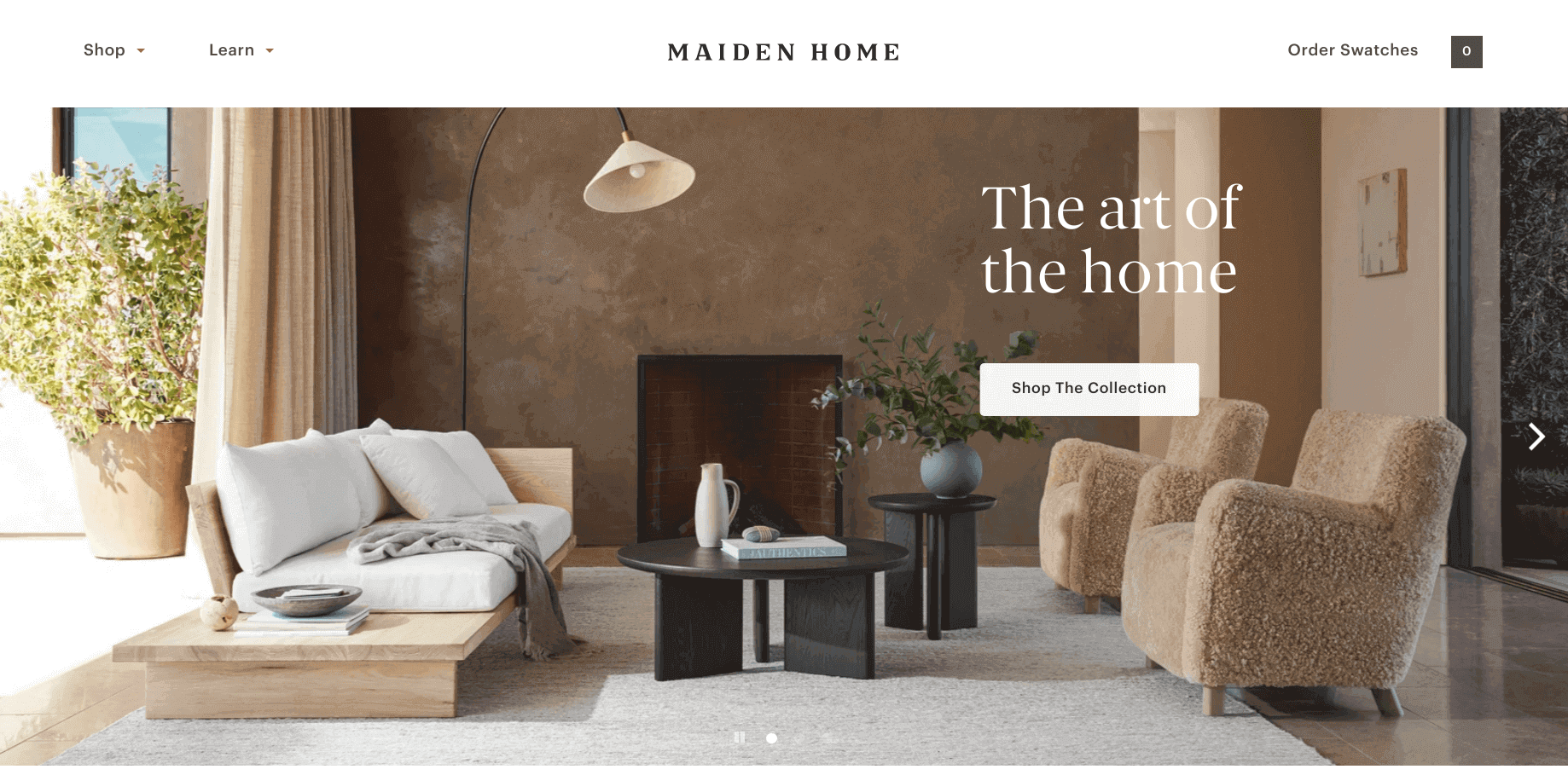This image showcases a webpage from the website Maiden Home, highlighting their elegant furniture offerings. The dropdown tabs labeled "Shop" and "Learn" are positioned in the top left corner, while the option to "Order Swatches" is on the right.

The centerpiece of the image is a modern living room with a sophisticated design. The room features two plush sitting chairs and a sectional sofa that has one open side. The coffee table and end table are both black and oval-shaped, creating a cohesive look. The coffee table is adorned with a vase, a rock, and a book, while the end table supports a flower pot with a thriving plant.

An additional table is integrated next to the open side of the sofa. The living room boasts a stylish decor, including a gray area rug on what appears to be a marble tile floor. The far wall, clad in brown galvanized steel, houses a sleek fireplace. A curved, minimalist lamp with a shaded single light bulb adds a touch of elegance to the space.

The right side wall features a photograph and what seems to be an entryway to another room. Behind the sofa on the left, there's a large curtain hinting at the presence of a sliding door. This area also includes a significant plant pot with a lush plant, through which sunlight gently filters into the room, enhancing its inviting atmosphere.